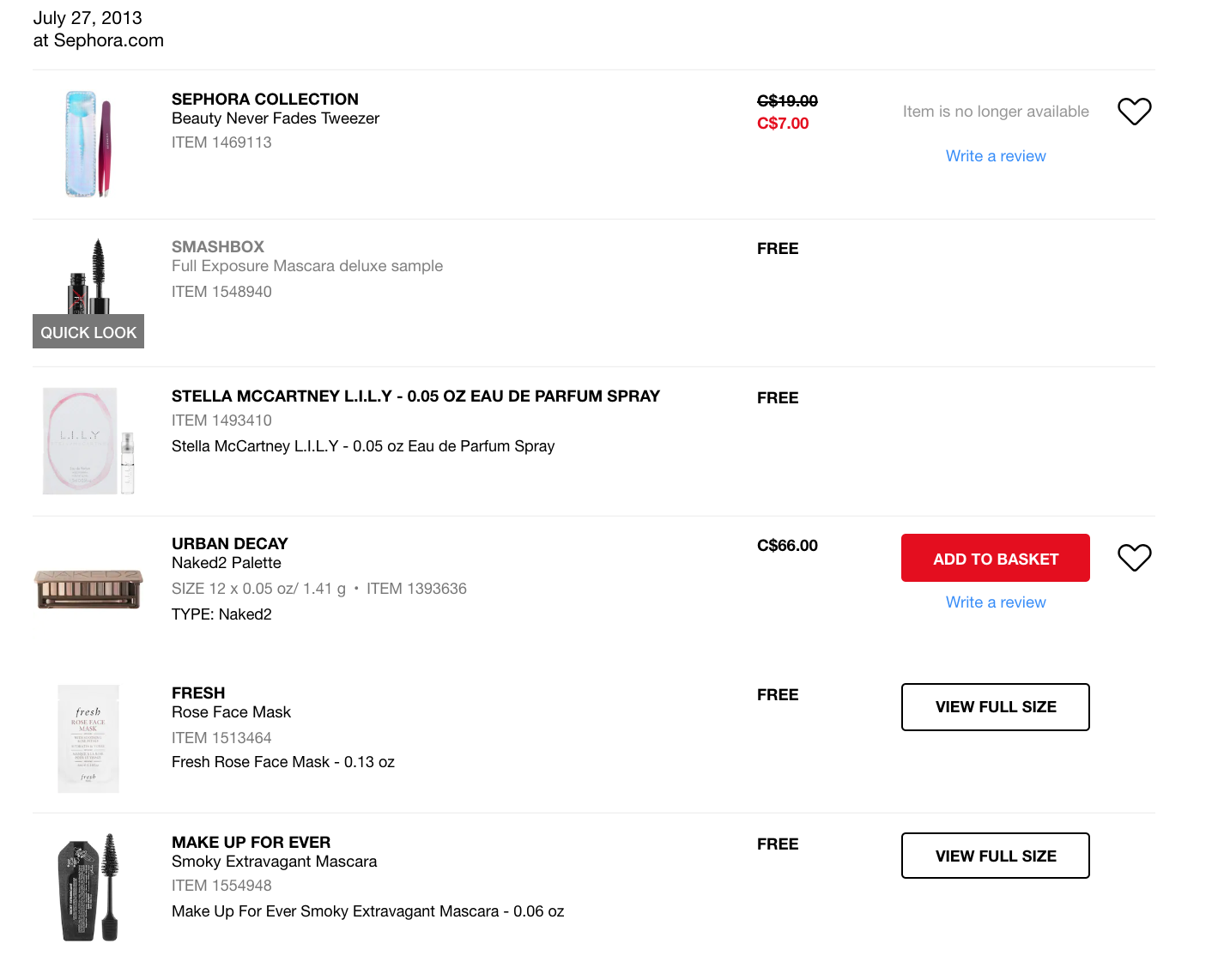This is an image of a webpage captured from Sephora's website on July 27, 2013. The webpage features a shopping cart summary, divided into six sections by faint gray lines for clarity. 

At the top of the page, there is the title indicating the website, "Sephora.com." The first item listed is the "Sephora Collection Beauty Never Fades Tweezers," accompanied by an item number and a note that it is currently unavailable. The tweezers are priced at CA$7 and are on sale. A blue section is visible for writing a review, and there is a heart icon to click if you love the item.

The second item is the "Smashbox Full Exposure Mascara Deluxe Sample," which is listed as free. Following that, the third item is also free and labeled as "Stella McCartney Lily Eau de Parfum Spray."

The fourth item is an "Urban Decay Naked 2 Palette" priced at CA$86, with an option to add it to the basket prominently displayed. 

The list also includes two more items, each with its corresponding image on the left, a detailed description on the right, and the price or availability options on the far right, completing the display of the user's shopping cart as seen on the webpage.